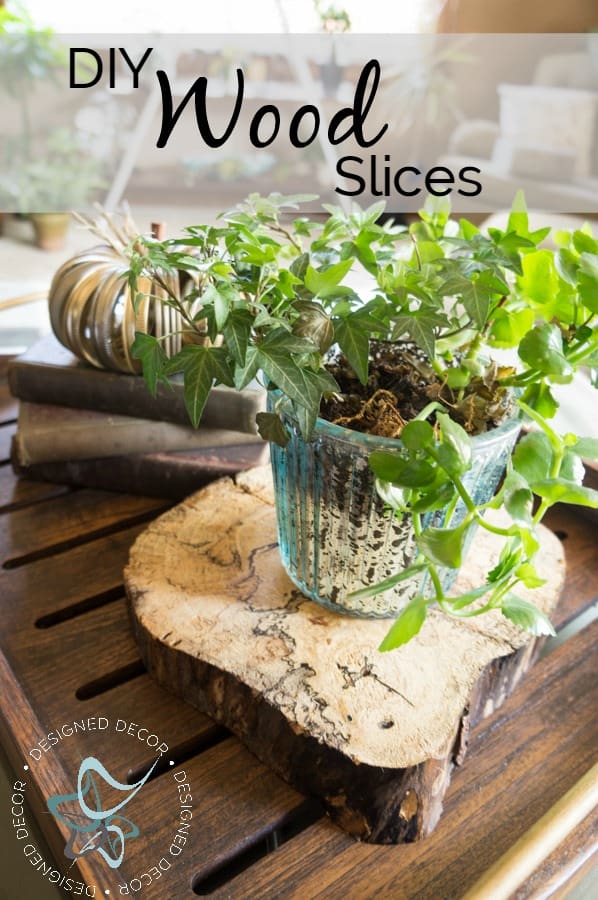The vertically aligned rectangular picture resembles a book cover for a how-to guide titled "DIY Wood Slices." The title is prominently displayed at the top in dark brown or black print, subtly emphasizing the instructional nature of the content. The letters "DIY" are in the upper left in capital letters, "Wood" is centrally placed below "DIY," and "Slices" is positioned to the right beneath "Wood," all set against a light gray rectangular backdrop.

The focal point of the image is the irregularly shaped slice of wood that serves as a base, resembling a piece of bread with its light brown top and dark brown bark-like sides. On top of this wood slice sits a fluted, round glass container, tinted blue, housing a lush houseplant. The plant, with green leaves and stems that fan out into three points, overflows the sides of the container. The wood slice and glass planter are placed on a dark brown wooden table featuring grooved cutouts.

Supplementing the scene is a circular logo in the lower left corner, composed of light blue and medium blue colors. The logo displays white text that reads "Designed Decor," repeating three times in a circular arrangement with white dots separating each repetition. The background reveals additional décor elements, including a metal pumpkin decoration and a hint of natural light filtering through a distant window, casting a soft ambiance over the entire setting.